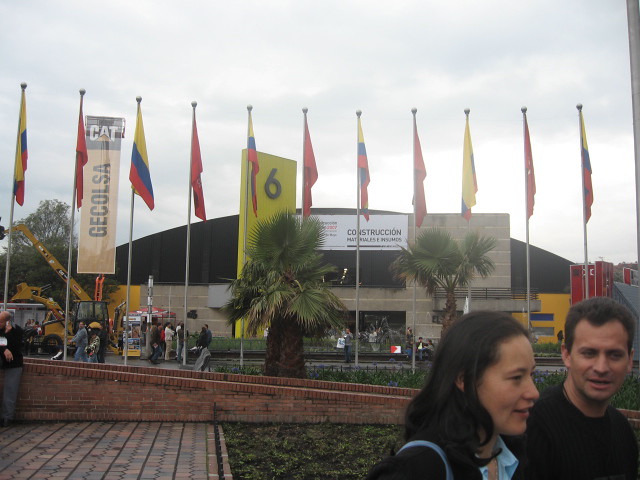In this photo, a middle-aged couple, both with dark brown hair and dressed in black shirts, stand outside under a partly cloudy sky. The woman has a baby blue strap on her left shoulder and a baby blue collar visible. They are positioned in front of a large beige building marked with the number six, which also features a line of about ten flags that hang still, indicating a lack of wind. Surrounding the couple are two palm trees, green grass, and a red brick walkway that runs through the scene. The area is bustling with people, suggesting a busy, perhaps public, location. Behind the couple, a crowd congregates near the building, with some individuals who appear to be construction workers. The building has a tan exterior and a black roof, further adding to the setting's detailed backdrop.